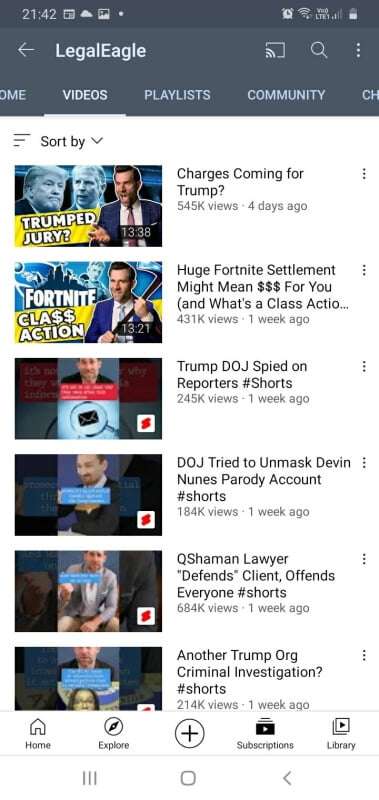The image appears to be a screenshot from a YouTube account, viewed on a mobile phone. The screenshot captures an overview of a YouTube channel that seems to focus on legal and political content, informally dubbed "Legal Eagle." At the top of the screen, there are tabs labeled "Home," "Videos," "Playlist," and "Community." A timestamp in the upper-left corner reads "21:42."

The "Videos" tab is prominently selected with bold lettering, showcasing a list of recent video uploads:

1. **"Charges Coming for Trump"** 
   - This video features a thumbnail with an image of Donald Trump alongside another individual labeled as "Trump's Jury."
   - It has garnered 545,000 views and was uploaded four days ago.

2. **"Huge Fortnite Settlement Might Mean Money for You"**
   - Accompanied by another video titled "What's a Class Action?"
   - The thumbnail includes the word "Fortnite" with the term "Class Action," where the 'S' characters are stylized as dollar signs ($).

3. **"Trump DOJ Spied on Reporters #shorts"**
   - This short video has accumulated 245,000 views over the past week.

4. **"Department of Justice Tried to Unmask Devin Noon's Parody Account #shorts"**
   - This video, featuring a man's image in the thumbnail, has achieved 184,000 views in one week.

5. **"Q Shaman's Lawyer Defends Client, Offends Everyone #shorts"**
   - This has a headlining count of 684,000 views in a week; the thumbnail showcases a man and a woman.

6. **"Another Trump Criminal Investigation #shorts"**
   - Garnering 214,000 views within the span of one week.

At the bottom of the screenshot, navigation options for "Home," "Explore," "Subscriptions," "Library," and a "+" sign are visible, indicating access to other parts of the YouTube app.